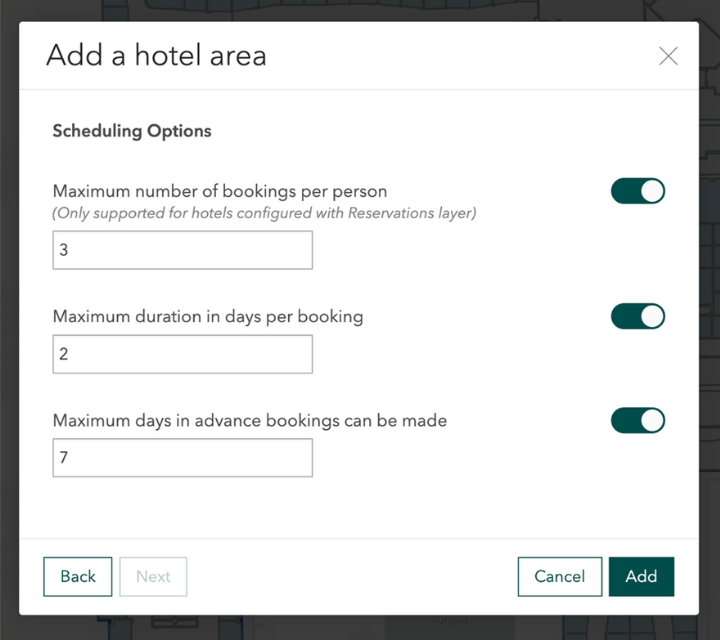The image depicts a structured interface with various sections and options related to hotel reservations, outlined by a black-bordered square. Within this black-bordered square is a smaller, centered white square. In the upper left corner, there is the label "Add Hotel Area" in black text. Below this, a thin gray line traverses the width of the square, and across the top section of the interface is a prominent gray 'X.'

Underneath the gray line, the text "Scheduling Options" is displayed in black. Following this, there's a space, and then the label "Maximum Number of Bookings Per Person" appears, also in black. Under this label, in gray text within parentheses, it reads "only supported for hotels configured with reservation letters layer."

On the right side of these texts, there is an oval with a part resembling a tail. Moving down, there is a left-aligned white rectangle with a black number '3' inside it. Below this rectangle, a second gray line stretches across the interface. 

Next, there is another label "Maximum Duration in Days Per Booking" in black text, followed by a similar white rectangle containing the black number '2', and another oval like the previous one. 

Continuing downwards, the label "Maximum Days in Advance Bookings Can Be Made" is visible, under which another white rectangle with the black number '7' is situated, accompanied by the same styled oval.

Towards the bottom of the interface, a final gray line cuts across the interface horizontally. On the left side is a pair of outlined buttons. The first button contains the text "Back" in teal font, and the second button, in a softer, less prominent style, reads "Next" in capital letters.

At the very bottom are two final buttons labeled "Cancel" and "Add".